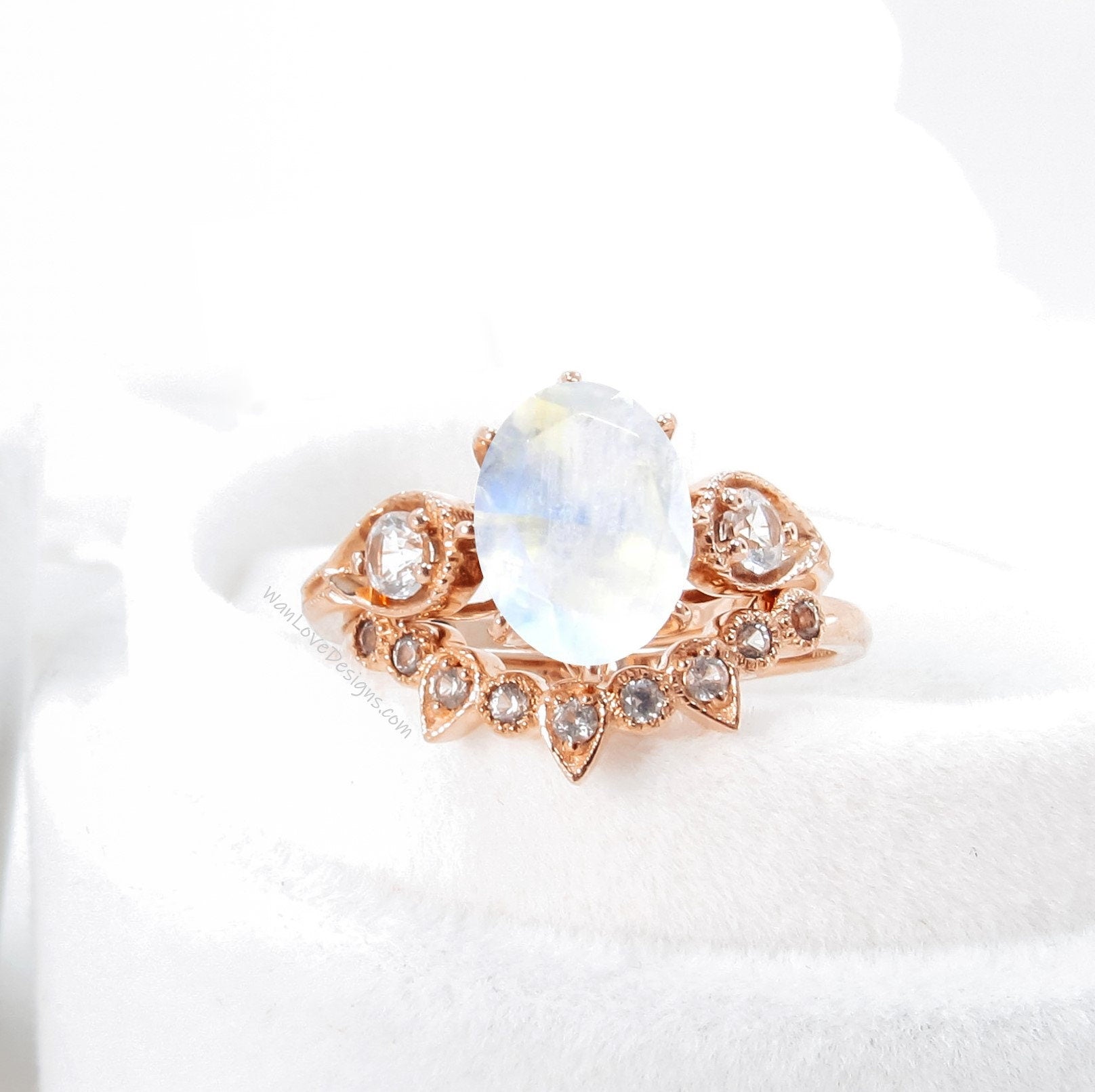The image features a golden ring displayed prominently on a solid white background. The ring is set inside a fuzzy, circular case that further accentuates its elegance. The band of the ring is gold and showcases a variety of sparkling gemstones, although their exact nature is somewhat ambiguous; they could be diamonds or rhinestones. The centerpiece is a large, smooth, oval-shaped gemstone that stands out due to its cloudy quality, suggesting it isn't finely faceted like typical diamonds. Flanking this central gemstone in a U-shape are two smaller circular diamonds. On the lower part of the band, a series of teardrop-shaped designs each enclose a small diamond, interspersed with singular circular diamonds, creating an intricate pattern, repeating "circle-teardrop" motifs. The case and background highlight the ring, making it the focal point of the image, with "Wayandlovedesigns.com" subtly visible in the scene.